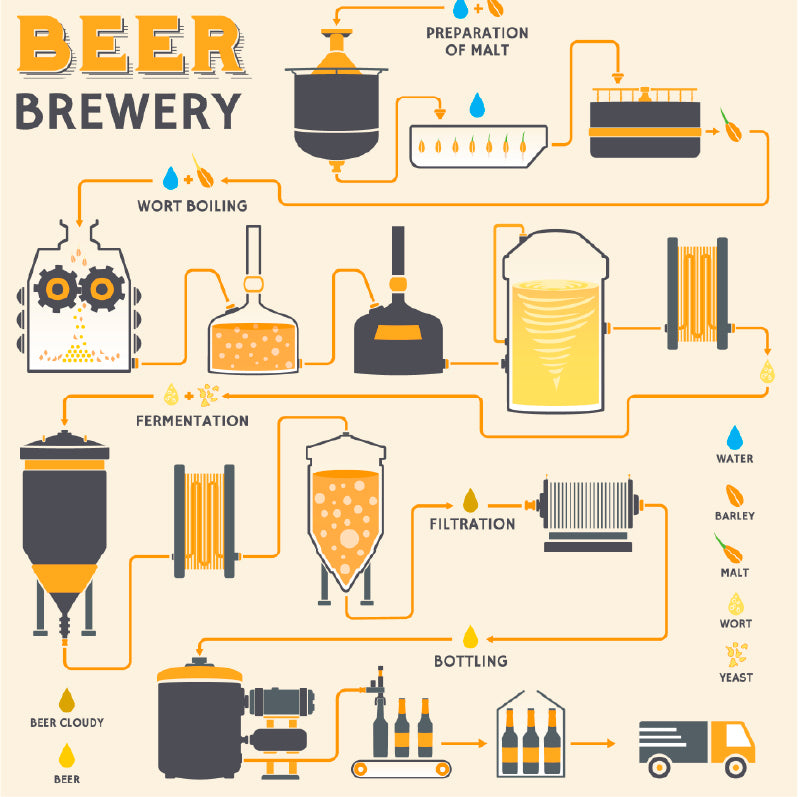This intricate diagram titled "Beer Brewery" at the top left corner showcases the detailed step-by-step process of brewing beer, starting from the preparation of malt to the final bottling and packaging. At the onset, it illustrates the "Preparation of Malt," symbolized by a drop, a bean, and arrows guiding the flow from a malt-prepping machine to a container indicating malt soaking. It transitions through various stages; next, it addresses "Wort Boiling," detailed with illustrations of sprouted beans and boiling flasks. Following an arrow path to fermentation, depicted by large containers, one transparent showing yellow liquid, and another opaque.

The filtration stage follows, represented by a black object with vertical lines, processing the liquid before leading to bottling. Bottling is depicted through a machine dispensing the liquid into tall bottles placed on a conveyor belt, followed by packaging and loading on a truck. Key aspects such as the ingredients (water, barley, malt, wort, and yeast) are listed on the bottom right, and the dark yellow "beer cloudy" and yellow "beer" drops are indicated to discern between stages of clarity in the beer production. The orange-highlighted arrows guide the viewer through each phase in this brewing journey, concluding with the finalized beer being prepared for distribution.